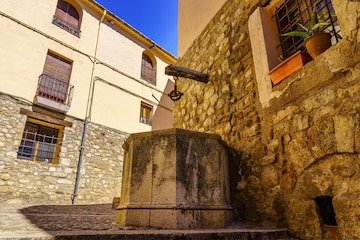This photograph captures a quintessentially European, likely Italian, scene with a strong Tuscan or Sicilian architectural influence. At the center of the small, outdoor image is an old water well, potentially fitted with a mechanism for lowering a bucket. The well, heavily shadowed, suggests minimal sunlight exposure and displays signs of age with possible mold on its stone panels.

The alley surrounding the well is paved with cobblestones, continuing the rustic charm into the street and building foundations. There are two main buildings, both showcasing a dual-style façade: the lower parts feature robust stonework while the upper sections are finished in cream-colored stucco.

In the background, a three-story building presents this combination with five visible windows. These windows are distinctive, rounded at the top and rectangular at the bottom. In the foreground, a similar building reveals a window adorned with potted plants, enhancing the visual appeal. Although the windows are fortified with bars, allowing space for potted plants, there are no walk-out balconies, only wrought iron railings.

A mix of functional and aesthetic elements like metal piping—possibly for drainage or electrical wiring—runs up the walls. Despite these practical features, the scene maintains a serene, old-world charm, reminiscent of a picturesque alley in a historical European setting.